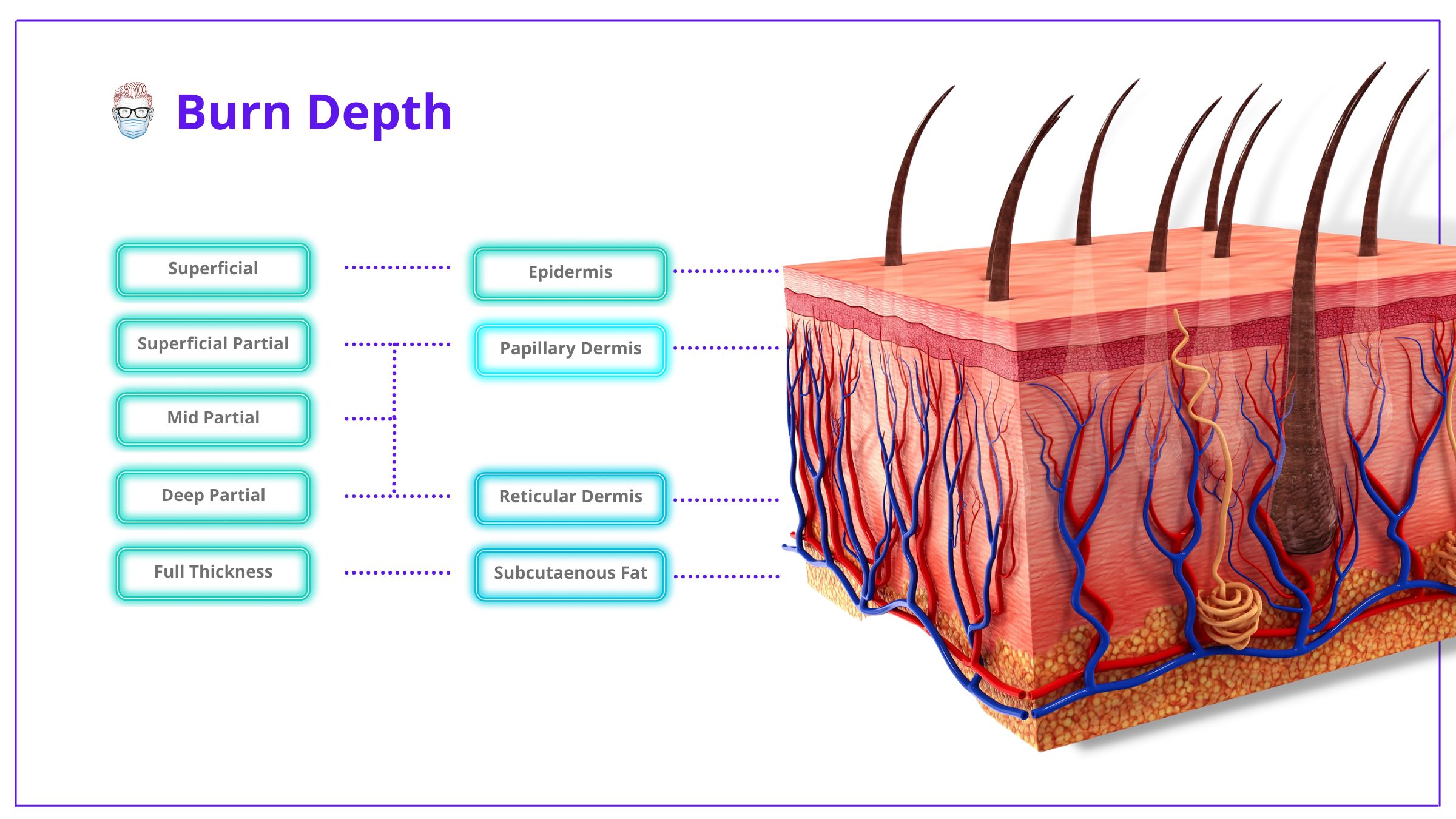The image is a detailed infographic on a white background, illustrating the burn depth classification of human skin in a cube-shaped, cross-sectional diagram situated on the right side. The upper left side of the infographic prominently features the title "Burn Depth" in purple text. Below this title, the layers of skin affected by burns are clearly labeled within turquoise rectangles with black text.

The infographic organizes the burn depths as follows: 
1. **Superficial** - Limited to the **epidermis**, represented by the pink topmost layer.
2. **Superficial Partial** - Affects the **papillary dermis**, shown as a red layer beneath the epidermis.
3. **Mid-Partial** - Not expressly detailed but implied to be between the papillary and reticular dermis.
4. **Deep Partial** - Reaches the **reticular dermis**, depicted as a deeper pink layer with visible blue and red veins and hair follicles.
5. **Full Thickness** - Extends down to the **subcutaneous fat**, illustrated as an orange, dotted area at the bottom of the cross-section.

Additionally, there's a visual representation of a person wearing glasses and a mask, reinforcing the clinical context of the diagram. The cross-section prominently includes features such as hair follicles protruding from the skin, blood vessels, and subcutaneous fat, with dotted lines aiding in the connection between the burn classifications and the corresponding skin layers.